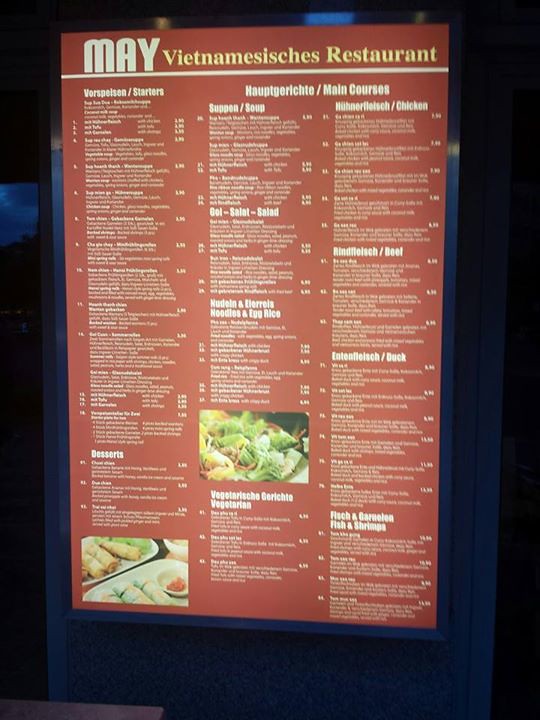This photograph showcases a restaurant menu set against a dark, nondescript background, emphasizing the menu as the primary focus. At the top left corner, the word "MAY" is presented in bold white font, accompanied by the phrase "Vietnamese Dishes Restaurant," indicating the establishment's specialty in Vietnamese cuisine. Despite the low resolution making most of the text illegible, certain sections are discernible.

In the upper portion, the term "Vorspeisen / Starters" is visible, followed by a list that presumably details the appetizer options. Below, the section labeled "Dessert" features a list of sweet treats, alongside a picture of egg rolls and spring rolls, suggesting popular choices.

The central part of the menu lists "Soupen / Soup" and "Goal Salad / Salad," highlighting the availability of soups and salads. Further down, the categories "Noodles and Egg Rice" and "Vegetarian / Vegetarian" are displayed, indicating options for noodle dishes, rice dishes, and vegetarian fare. A picture of a salad accompanies these sections, providing a visual aid.

To the right, headings such as "New Chicken / Chicken," "Beef," "Eletelflesk / Duck," and "Fish and Garum / Fish and Shrimps" are visible, suggesting a variety of protein-based dishes. The entire menu features a red background with white font, enhancing readability and adding a vibrant touch.